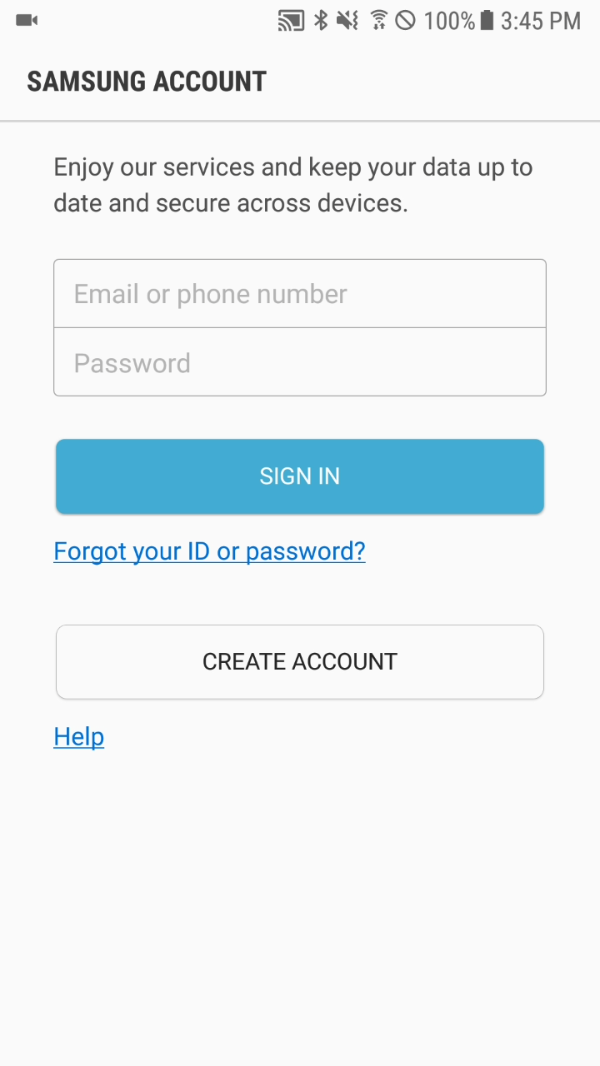This image is a mobile screenshot taken from a Samsung device, likely running on an Android platform. The screenshot is in a tall rectangular format, showing the device's status bar at the top. The time displayed is 3:45 PM, and the device has a full battery and a strong Wi-Fi signal. The audio is muted, indicated by a speaker icon with a slash through it. The Bluetooth feature is active, signified by the Bluetooth icon, and the device appears to be casting or mirroring its screen, as shown by an icon resembling a screen with a Wi-Fi signal.

The main content is a white background page displaying the Samsung account login interface. At the top, in bold black text, it reads "Samsung account," followed by a horizontal line. Beneath the line, the text prompts, "Enjoy our services and keep your data up to date and secure across devices." 

Two input fields are visible: the first is for entering an email or phone number, and the second is for the password. Below these fields is a prominent blue "Sign in" button with white text. Additional options include a link for users who have forgotten their ID or password and a white "Create account" button with black text. Below this button, there is a help link for further assistance.